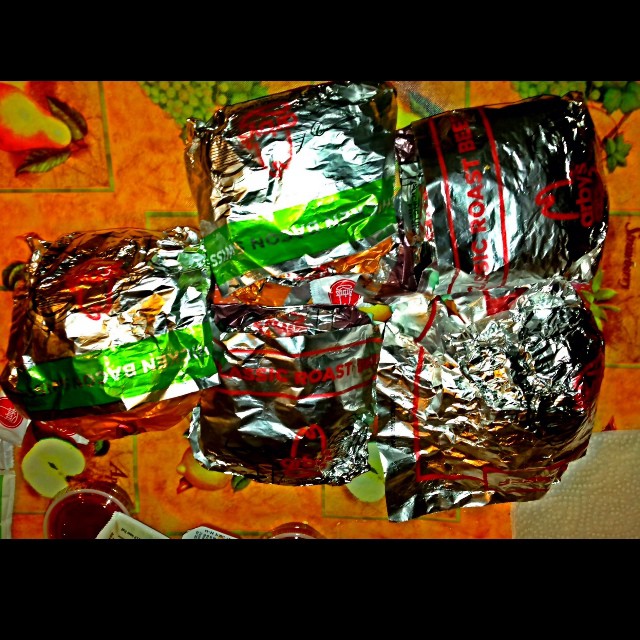This top-down photograph captures five poorly wrapped sandwiches from Arby's, identifiable by the red Arby's logo on their highly reflective silver foil wrappers. Two of the wrappers feature horizontal green lines, indicating they are "Bacon Swiss" while others appear to be labeled "Classic Roast." These sandwiches are laid out on a table draped with an orange tablecloth adorned with a colorful fruit pattern, including grapes, pears, peaches, and apples. The scene is illuminated by harsh light, causing extreme reflectivity from the silver wrappers which makes the text difficult to read. A cheap, white paper napkin and several small plastic containers of dipping sauces, possibly for barbecue or ketchup, are situated nearby, adding to the casual, fast-food presentation.